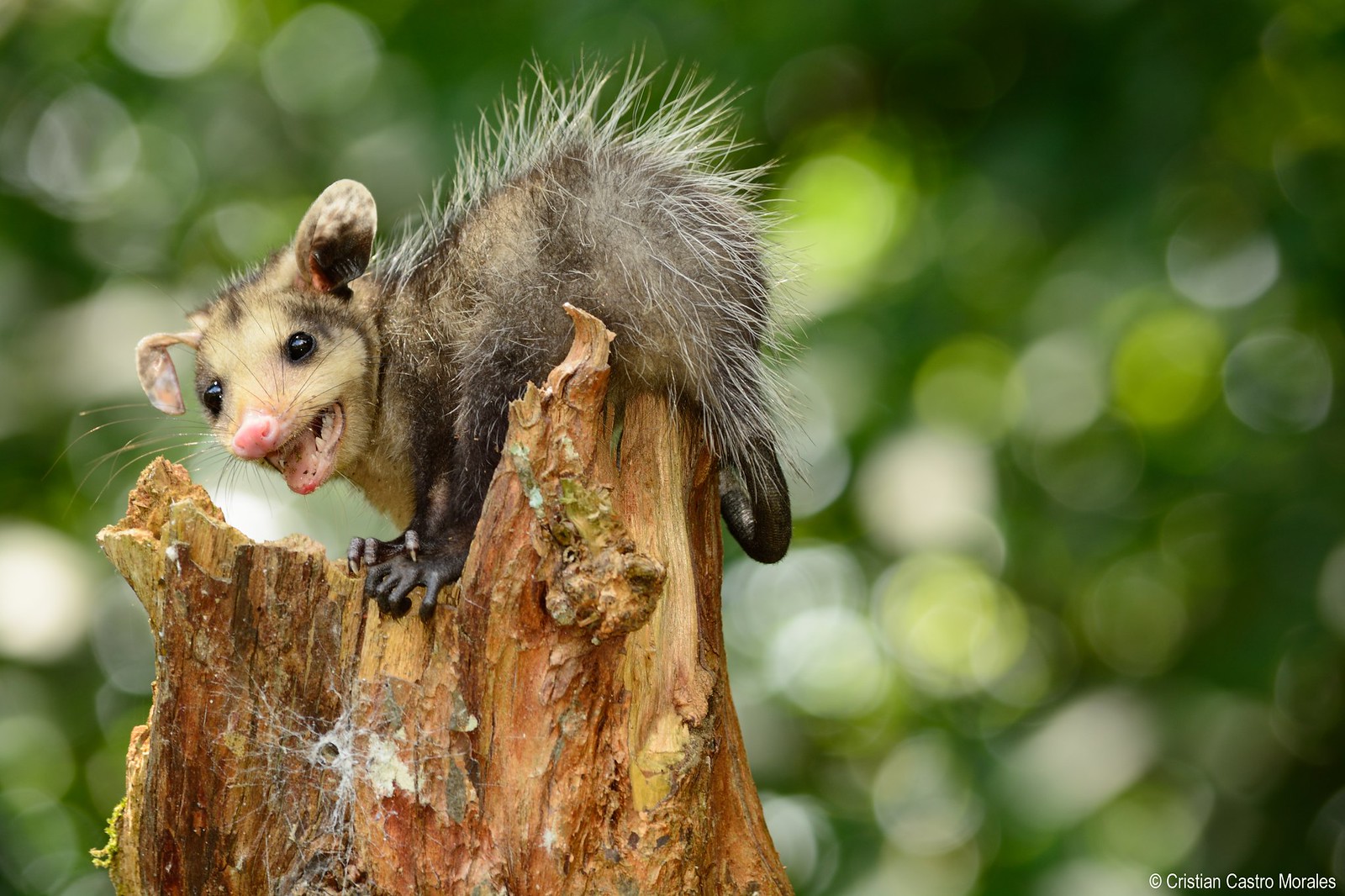In this photograph, taken outdoors with a blurred background hinting at trees and various shades of green, a baby possum is the focal point. The rectangular image captures the possum perched on a jagged, broken log, possibly an old tree stump, adorned with spider webs. The baby possum, displaying a mix of beige and darker coloration on its legs and tail, clings to the log with its little hands while its tail and feet hang off the back. Facing the camera with an open mouth that reveals a pink nose and tongue, the possum gives an impression of vulnerability and possibly being underfed. Several long, white hairs sprout from its body, adding to its delicate appearance. Despite its endearing qualities, the possum's small size and open mouth give it an almost sinister, yet inexplicably captivating presence.